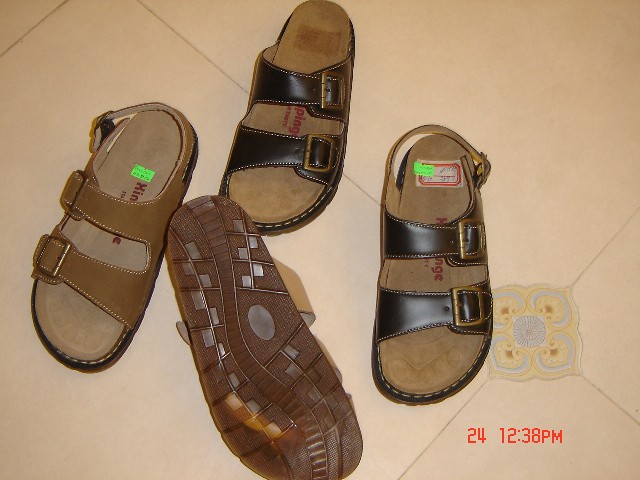The image features a beige tiled floor with intricate gold and light blue floral designs at the intersections where the four tiles meet. In the bottom right corner, a red timestamp reads "24, 12, 38 p.m." Centered on the floor, four Birkenstock-style sandals are arranged in a rough circle. The sandals are of various shapes and colors: two are dark brown, and two are mid-brown, each with two straps with brass buckles and stitching along the edges. Two sandals include a back strap. The sandals, described as having a wide, beige suede footbed, one of which is flipped over to reveal a map-like tread pattern with sections of rectangles, triangles, and an oblong circle. The shoes are new, sporting green neon sale stickers over their original price tags.